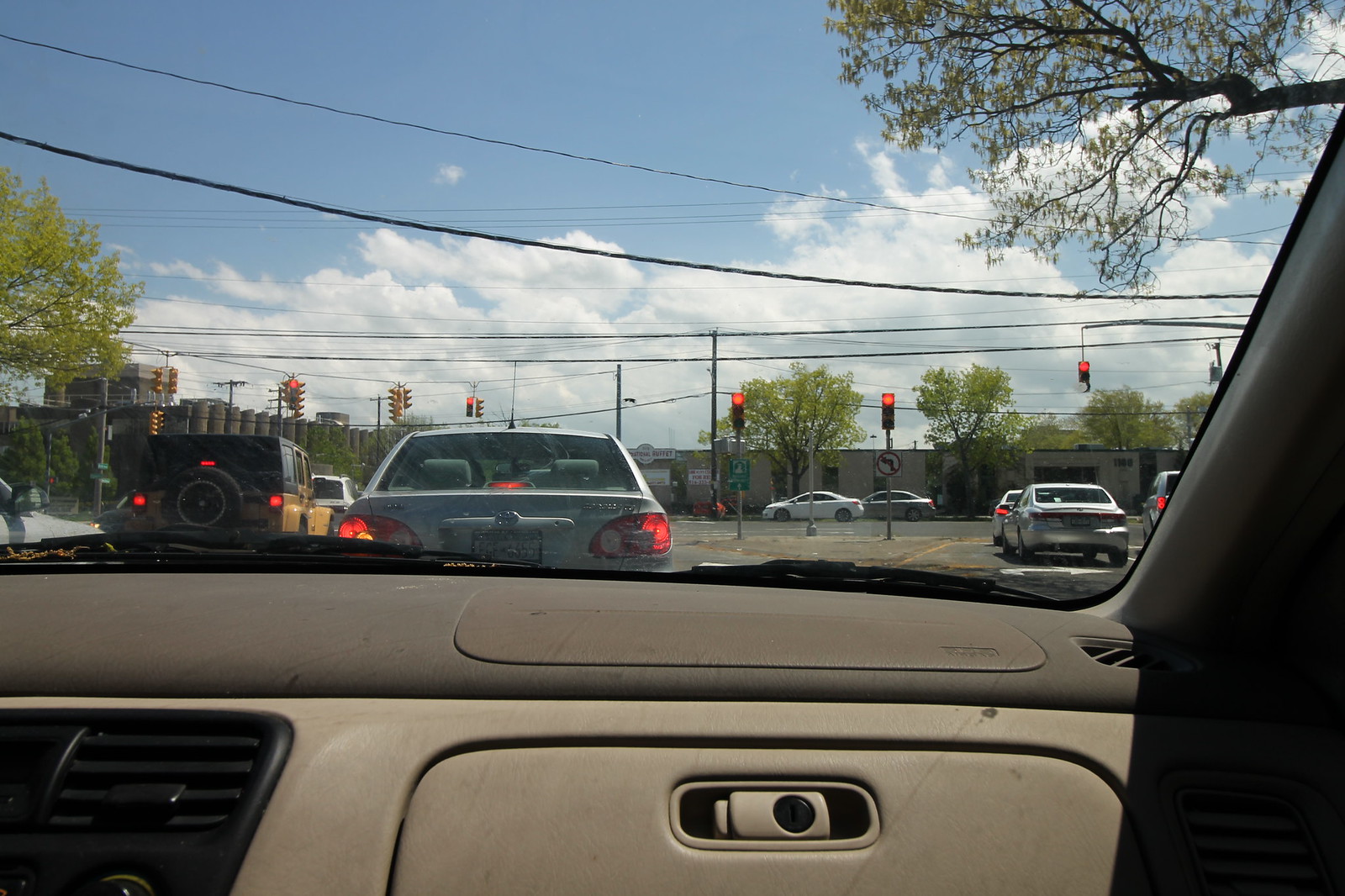This daytime photograph captures the view from inside a vehicle, showcasing a partial glimpse of the tan and dark gray interior, including the glove box. Through the windshield, a clear blue sky with fluffy white clouds can be seen, punctuated by overhead black power lines. The scene also features several leafy green trees. The street ahead is bustling with varying vehicles, including silver cars with illuminated taillights, a distinctive gold Jeep with a black top, and additional white and gold cars. Multiple traffic lights are visible, several glowing red, alongside a no-turn sign with red markings and a green sign mounted below one of the stoplights. The overall image quality is remarkably clear, providing a detailed snapshot of this urban scene.